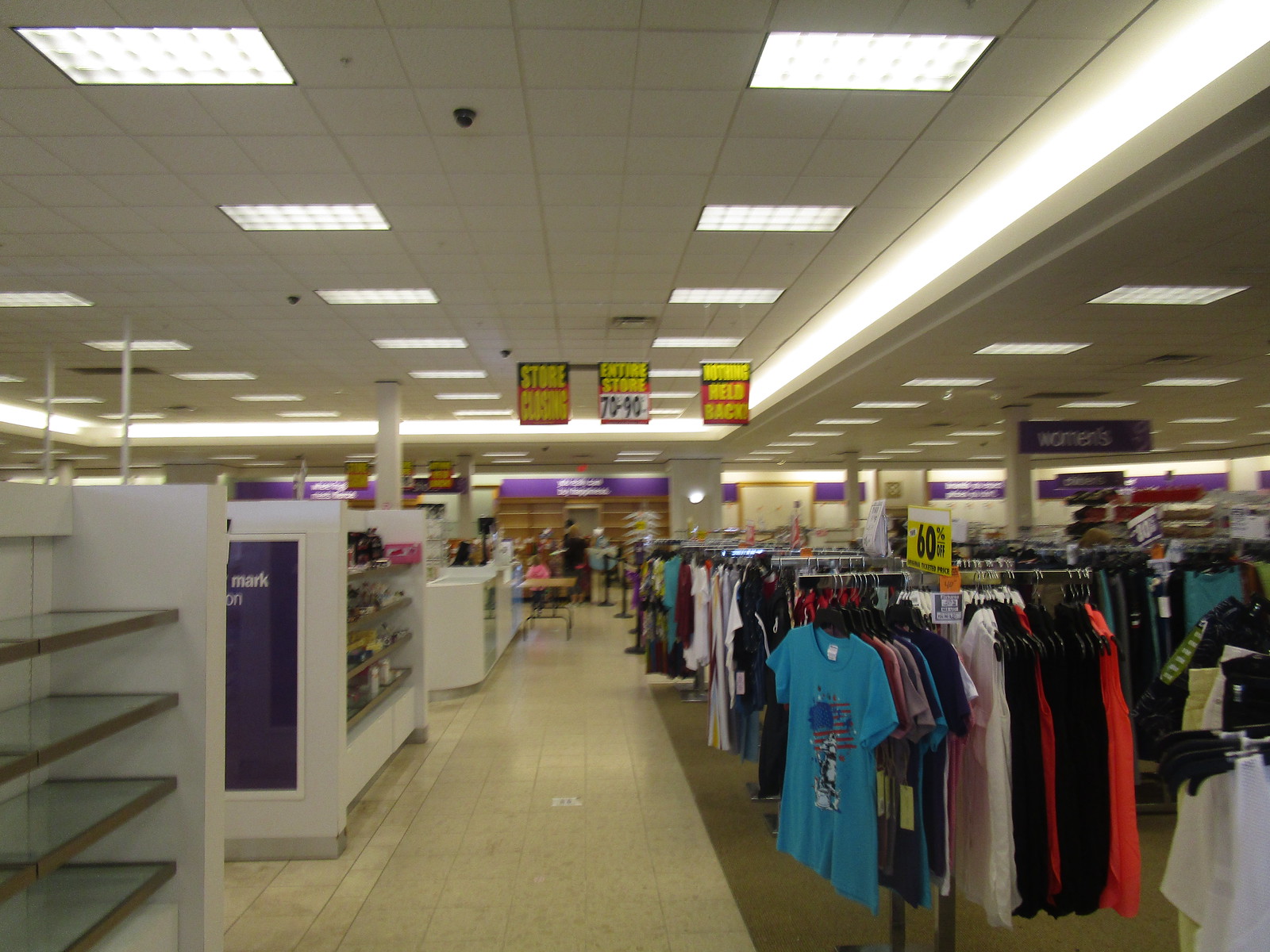The image depicts the interior of a plain, nondescript clothing store that is going out of business. The store has a grid of white ceiling tiles, rectangular fluorescent lights, and a yellowish-white tiled floor with gray grout. As you walk in, you notice a mix of sparsely stocked and bare white shelves on the left. On the right, you see clothing racks displaying various items, including blue, red, white, and black t-shirts and women’s clothing, which are discounted at 60% off. 

Prominent black, red, and yellow signs hang from the ceiling. The sign on the left reads "Store Closing," the one in the middle announces "Entire Store 70% to 90% Off," and the one on the right says "Nothing Held Back." A brown carpet is visible in some areas, particularly under the women’s clothing racks. Further into the store, which has purple awnings in the back, more bare shelves are evident. The detailed discount signage and the state of the inventory underscore the final sale efforts before the store permanently closes.